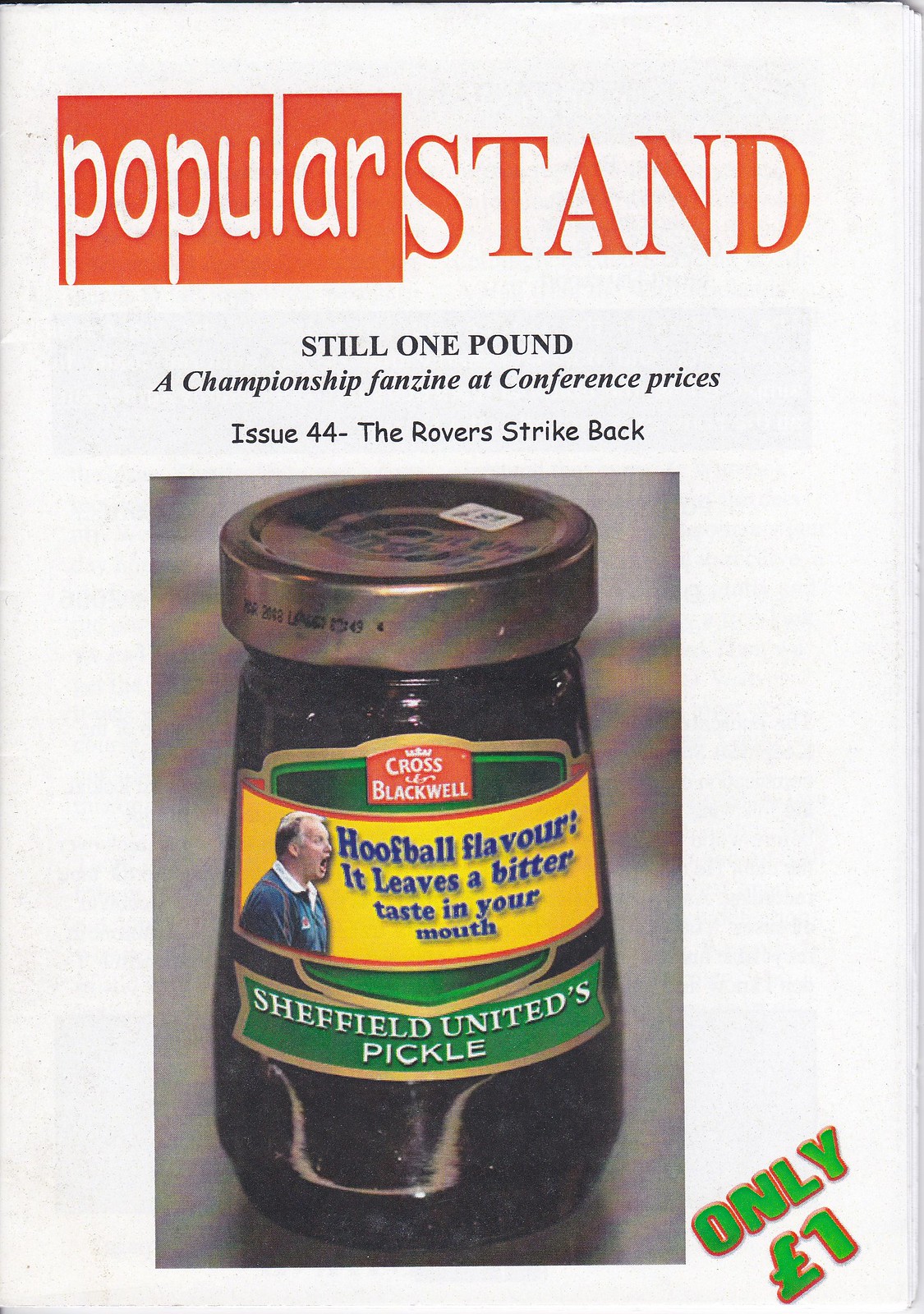The image is the cover of a fanzine with a primarily white background. At the top, there's a red rectangular area with the word "POPULAR" in white text. To the right, on the white background, red letters spell "STAND." Beneath this, in black text, it reads "STILL ONE POUND." Following this is the phrase "A Championship Fanzine at Conference Prices," also in black. Centered beneath that, the cover declares "ISSUE 44: THE ROVERS STRIKE BACK."

Dominating the middle portion of the cover is an image of a black jar with a bronze-colored screw-top lid. The label on the jar features the brand name "CROSS BLACKWELL" at the top. An illustration of a man shouting is placed to the left side of the label, and next to him, the text "HOOFBALL FLAVOR" is prominently displayed with the tagline "It leaves a bitter taste in your mouth." Below this, it states "Sheffield United's Pickle." Finally, on the bottom right corner, angled in green text, it reads "ONLY ONE POUND," which may also appear as "ONLY ONE EURO," indicating its appeal to a broader audience.